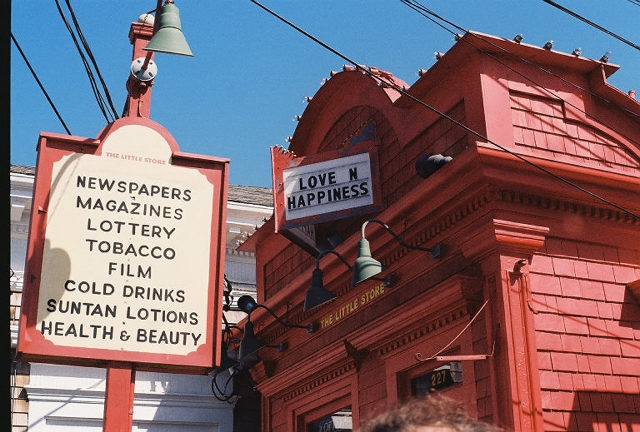This photograph captures the exterior of an antiquated building, reminiscent of an old-timey establishment. The structure exudes a nostalgic charm, decidedly different from modern architecture. It features a facade bathed in striking, bright red hues that are uncommon in contemporary storefronts. The design hints that it could be a historic theater or perhaps a quaint candy store.

To the left side of the building, there is a tall, narrow red sign with a beige background and black text detailing the store's offerings. The vertically arranged list reads: **newspapers, magazines, lottery, tobacco, film, cold drinks, suntan lotions, health and beauty**—suggesting that this is an all-in-one store catering to a wide variety of needs.

Above the entrance, a prominent sign reads "Love and Happiness," imbuing the building with a sense of warmth and inviting sentiment. This quaint yet vibrant storefront evokes a sense of nostalgia and community spirit through its vivid colors and diverse array of products.